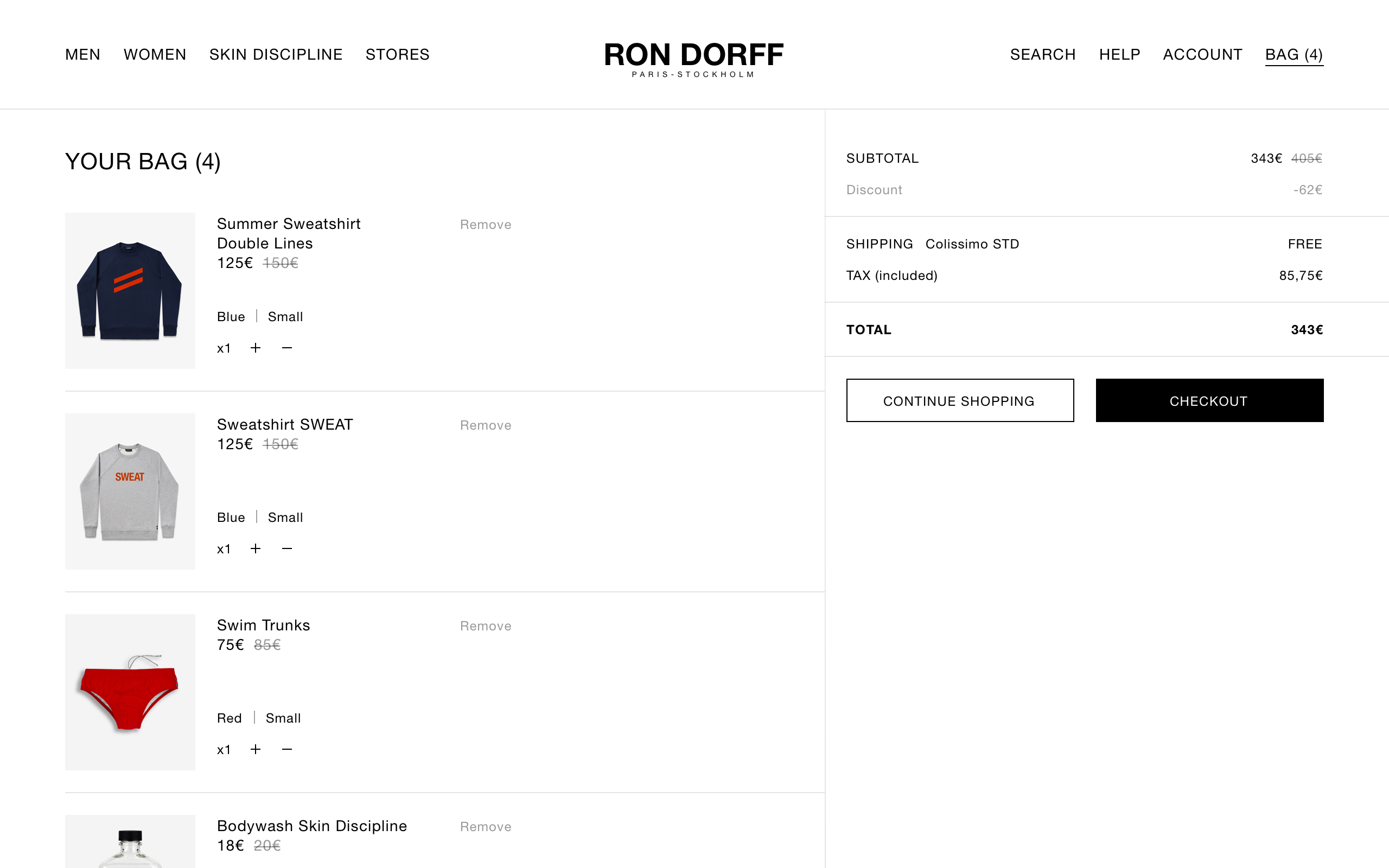In this rectangular image set against a solid white background, we see a screenshot of a shopping website. At the top center, the business name is prominently displayed in bold black text: "Ron Dorf, Paris, Stockholm." Located in the lower left corner, stretching from left to right, are navigational options labeled: "Men, Women, Skin Discipline, Stores, Search, Help, Account, Bag, For."

On the left side of the image, there is a vertical section labeled "Your Bag." The first item listed is a "Summer Sweatshirt," priced at 125 units of currency which appears to be Euros (€). Below this sweatshirt, in blue text, the size is denoted as "Small." The next item is a pair of red bikini swim trunks, also in size small. Listed third is "Body Wash" from the Skin Discipline line, priced at 18 units of currency. The total amount for the items in the bag is 343 units of currency.